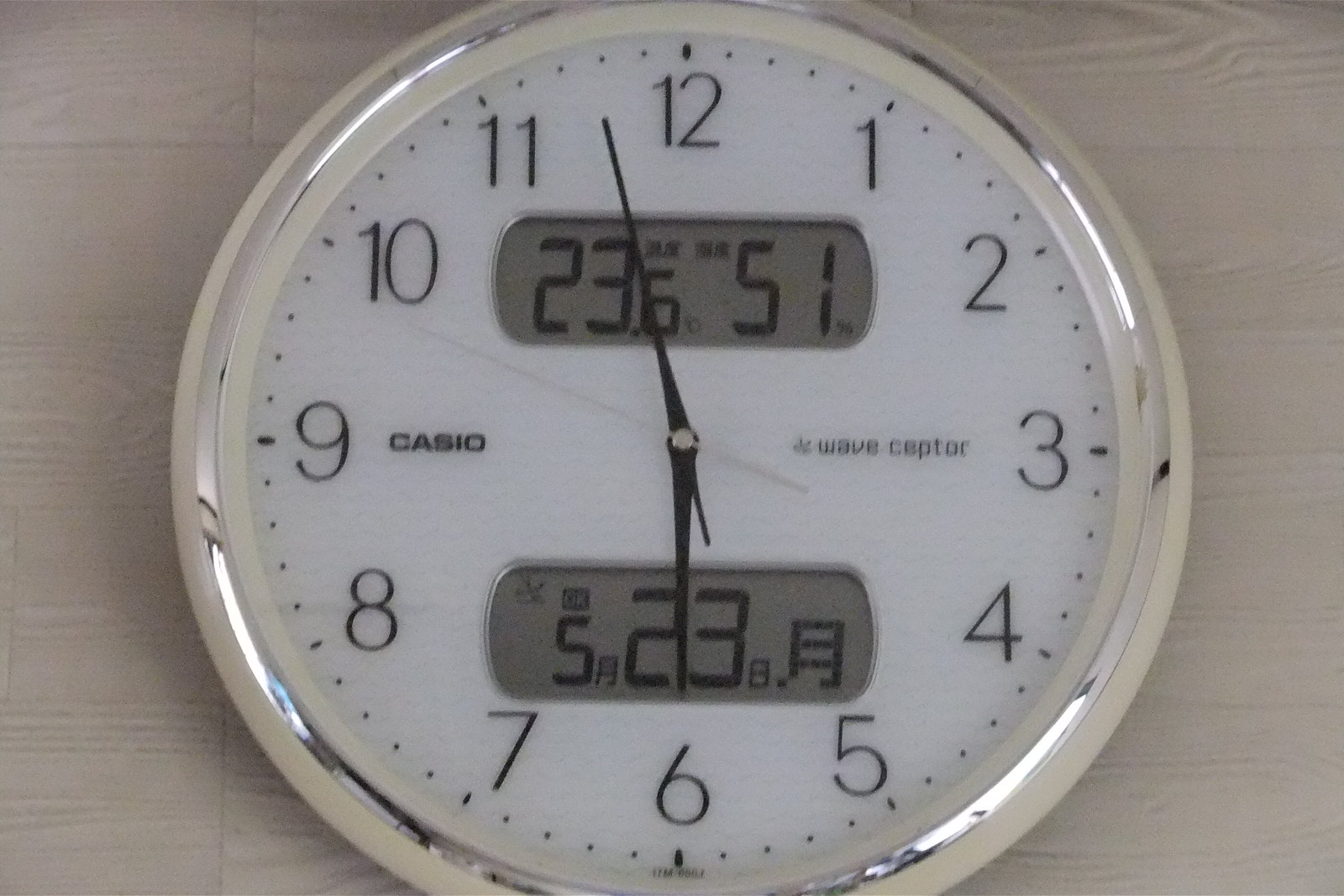A captivating photograph features a contemporary wall clock resting on a light wood-paneled floor. The backdrop of the image showcases the intricate grain of the light grey or dark cream-colored wood, adding a subtle texture to the scene. The clock, partially cut off at the top and bottom by the frame of the photo, exhibits a sleek silver chrome rim that complements its minimalist design. The clock face is pristine white, contrasted by bold black numerals ranging from 1 to 12. Centered on the face are black hour and minute hands, accompanied by a refined silver second hand. 

Adding to the modern aesthetic, the clock incorporates two digital panels: an upper panel displaying "23.651" and a lower one reading "523A," with varied font sizes to draw attention. On the left side of the digital displays, the brand name "Casio" is prominently featured, while the right side reads "Wave Captor," indicating its advanced functionality. Despite these technological elements, the clock maintains its classic appeal, blending tradition with contemporary design elements seamlessly.